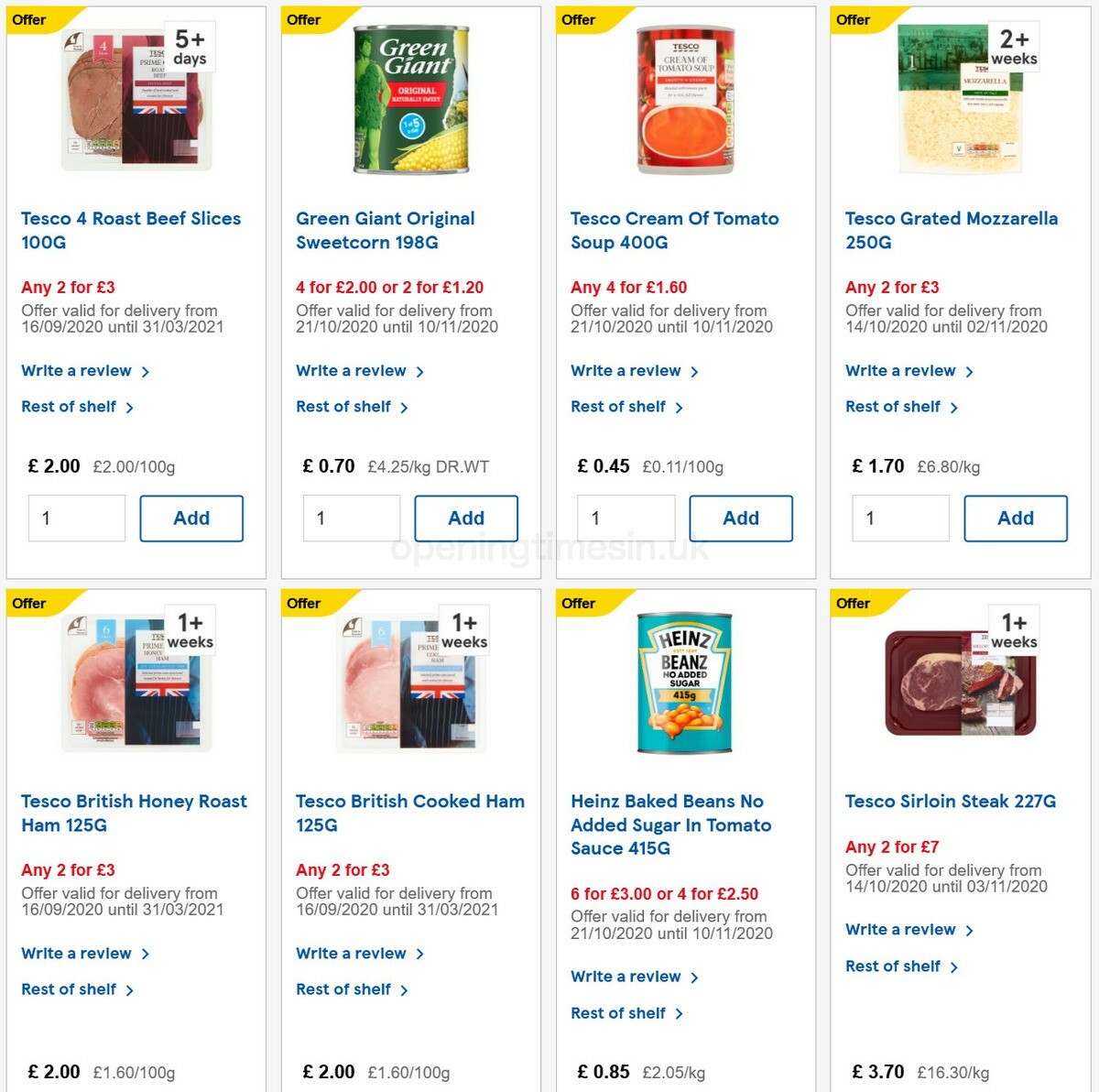Here is a refined and detailed caption for the image as described:

---

The image is a screenshot taken from a laptop displaying a shopping page on a grocery website in landscape mode. The layout consists of two rows and four columns, each separated by faint grey lines on a predominantly white background.

Each block within these rows represents an individual food item and is uniformly structured as follows:

- **Top Section**: Each block begins with an image of the product.
- **Item Identification**: Directly below the product image, the item name is featured in blue text.
- **Promotional Offer**: If applicable, a promotional offer is stated beneath the item name in red text.
- **Product Description**: Below the promotional text, a short description of the item is provided in black font.
- **Review and Shelf Information**: Two options in blue text - "Write a Review" and "Rest of Shelf" - are listed next.
- **Pricing Information**: The item's price is presented in bold black text, followed by the unit price.
- **Quantity and Purchase Options**: At the bottom, there is a quantity selection option and an "Add" button in teal located to the right.

Specific example from the upper left-hand corner of the image:

- **Offer Badge**: The upper left corner includes a yellow background label indicating a special offer.
- **Product Image**: Below the offer badge, there is an image of the product tagged with "5+ days" to indicate freshness.
- **Product Title**: In blue text, "Tesco Finest Roast Beef Slices 100g" is written.
- **Offer Details**: The offer details read "Any 2 for £3" with the valid delivery dates from 16/09/2020 until 31/03/2021 in red text.
- **Review and Shelf Links**: Below, it reads "Write a Review" and "Rest of Shelf" in blue text.
- **Price Information**: The price is shown as "£2" in bold black text followed by the unit price "£2 per 100 grams."
- **Purchase Button**: A blue button on the right side provides the option to add the item to the cart.

The bottom right corner similarly displays a different product, such as "Tesco Finest Sirloin Steak," with relevant promotional offers and purchase details well-organized in the same format, detailing any 2 for £7 deals.

---